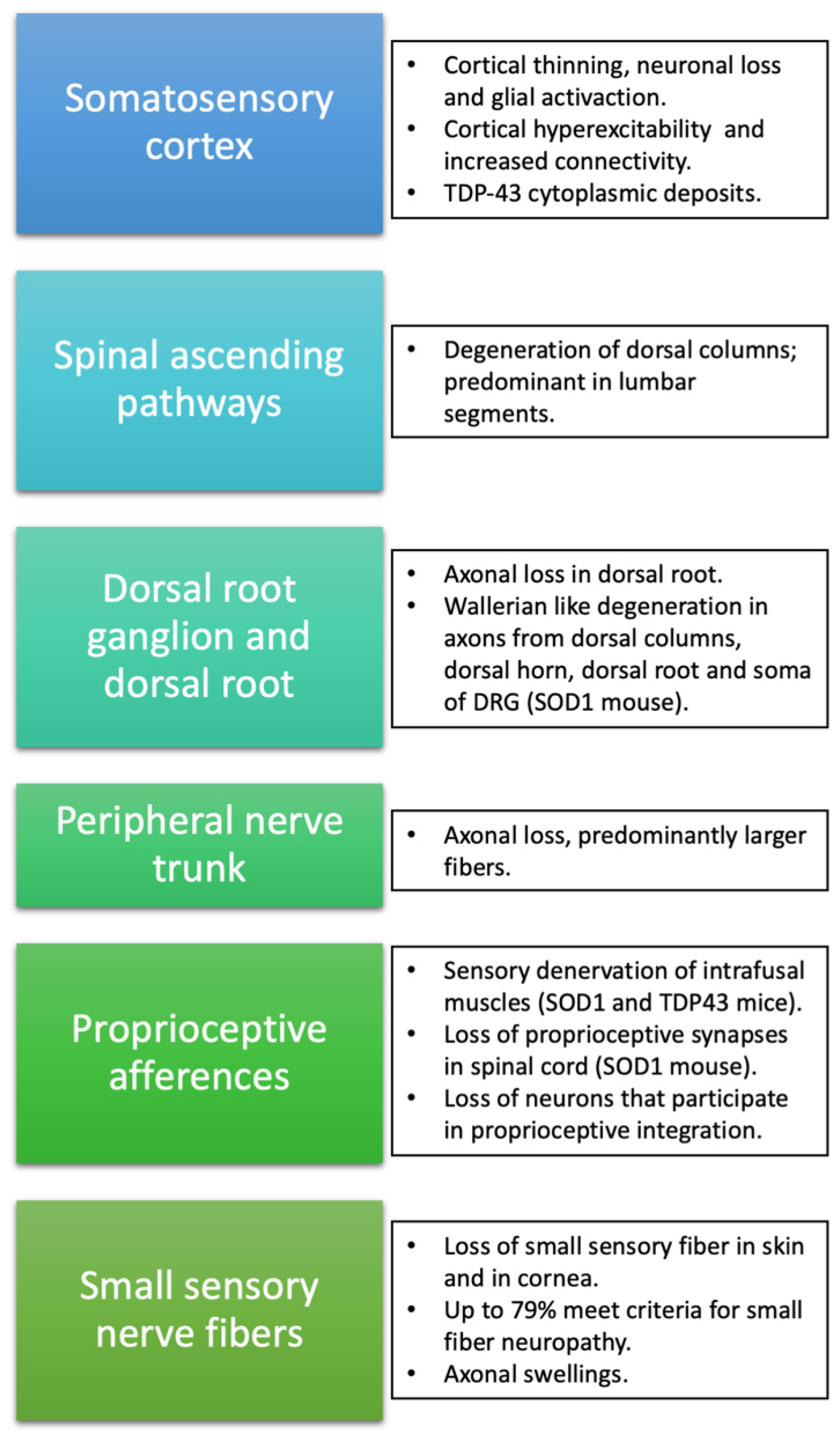This is an informational poster likely intended for medical students, detailing various components of the human neural pathway. The poster is divided into two vertical columns. On the left, six main points are highlighted in color-coded boxes that range from dark blue at the top to dark green at the bottom. These points include: somatosensory cortex, spinal ascending pathways, dorsal root ganglion and dorsal root, peripheral nerve trunk, proprioceptive afferences, and small sensory nerve fibers. Each of these main points is presented in white text on their respective colored backgrounds, creating a gradient effect from blue to green.

On the right side, adjacent to each colored box, are rectangular boxes with white backgrounds and black outlines. These contain detailed explanations of the main points, each box featuring between one to three bullet points. These explanatory notes cover topics such as cortical thinning, neuronal loss, and glial activation. The overall layout positions these descriptive boxes directly beside the colored boxes, visually aligning the explanations with their corresponding neural components. The poster's clean design and organized structure make it a useful educational tool for understanding the somatosensory neural pathways.